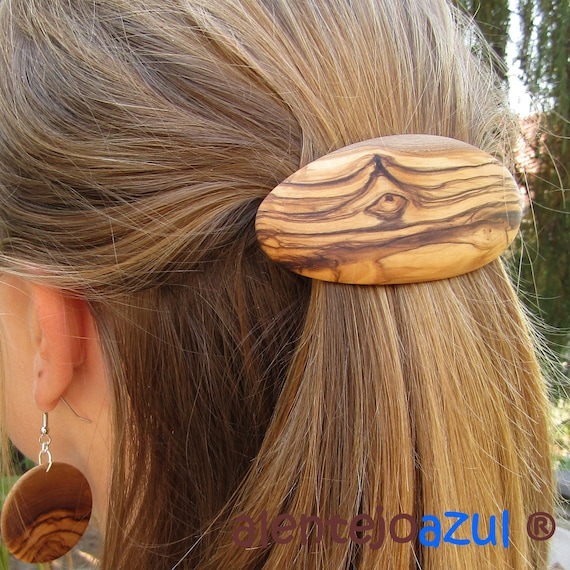This photograph focuses on the back of a woman's head with longish chestnut brown hair intertwined with subtle blonde highlights. Her hair is styled into a ponytail held securely by an oval-shaped wooden barrette, which shows off decorative dark brown and golden wood grain highlights, lending it a slightly dull but finished appearance. Dangling from her left ear is a round wooden earring that matches the barrette, adding to the cohesive look of her accessories. The woman has fair skin, and the backdrop consists of tall, green, coniferous shrubs, suggesting an outdoor setting. At the bottom of the image, there’s a watermark overlay with the text "O-LEN-J-NA, O-LEN-J-NA, O-LEN-J-NA, O-LEN-TE-HO" in brown and "Azul" in blue, alongside a circled "R" symbol, likely indicating a brand or trademark.